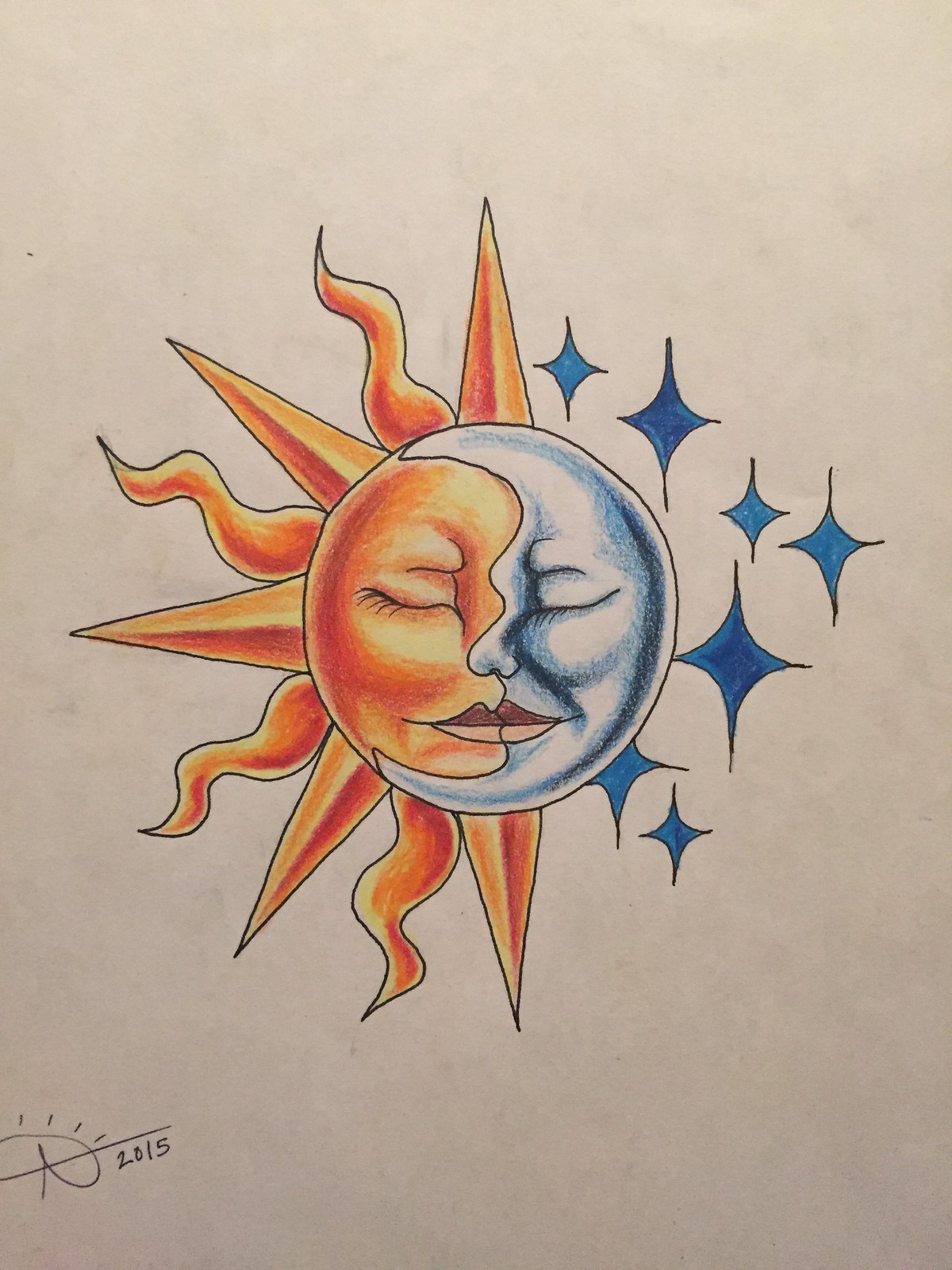This is a color photograph of an illustration depicting a half sun and moon combination. The drawing is on a sheet of paper with a greyish-beige hue, potentially due to the lighting. The left side of the illustration represents the sun, featuring orange and yellow triangular shapes and squiggly lines extending outward like rays. The right side symbolizes the moon, rendered in bluish-grey hues with dark blue stars made of inwardly curved lines with points instead of spikes.

Both celestial bodies share a central circle that forms a human-like face with closed eyes. The facial features are cleverly designed to be either viewed independently or as part of a single cohesive face, creating a dual perspective. The sun and moon share one eye on each side and a set of lips in the middle. The illustration is signed in the lower left-hand corner with what appears to be "R or P, 2015." The overall image has slight textures or smudges, adding a tactile quality to the artwork.